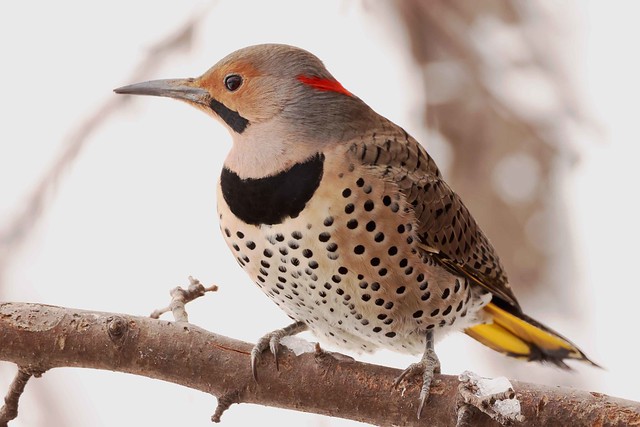The photograph captures a detailed winter scene in a snowy woodland area, with a blurred, white background that accentuates the cold, serene ambiance. Dominating the foreground is a small, gray-brown branch stretching horizontally from right to left, adorned with tiny offshoots. Perched centrally on this branch is a bird, exhibiting a striking array of colors and patterns.

The bird's face features a vibrant orange area around its eyes, a distinguished gray head, and a prominent red stripe diagonally across the back of its neck. Its long, slight curve of a gray beak points to the left, in the same direction as its gaze from a single, visible black eye. The bird's throat sports white feathers, transitioning to a distinct black crescent shape on its breast, which continues as a multitude of black spots dotting its light brown chest.

Further details reveal the bird's wings adorned with gray and brown feathers interspersed with additional black spots. Its tail feathers, extending downward to the right, are marked by both light and dark yellow hues. The bird’s talons and feet, which clutch the branch securely, are a combination of gray and yellowish tones. This vivid and diverse plumage stands out against the blurred, snowy backdrop, making the bird the clear focal point of the image.